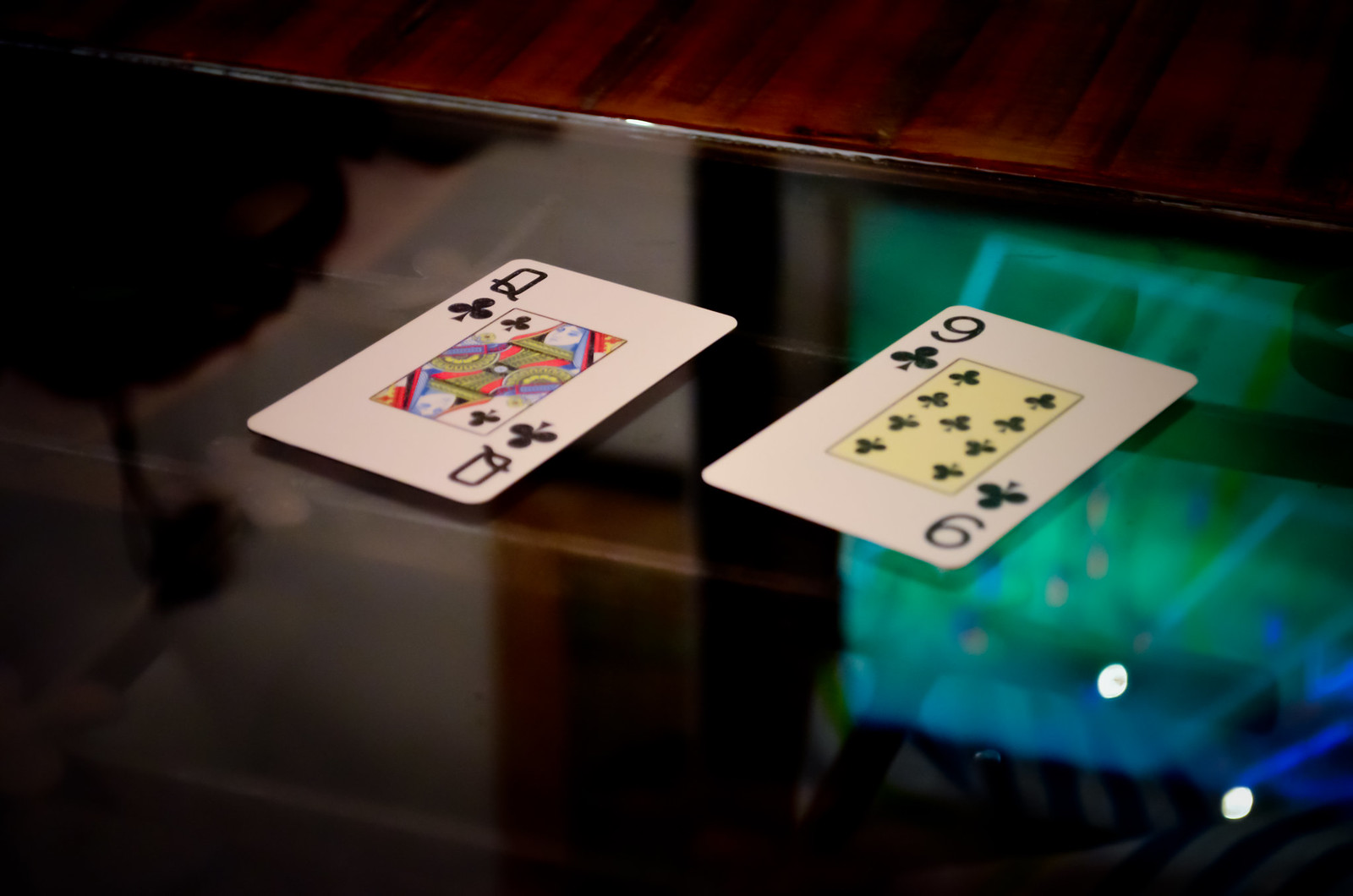Two standard-sized playing cards, the Queen of Clubs and the Nine of Clubs, are placed side by side on a pristine glass table. The cards are oriented on a slight diagonal, with a small space separating them. The glass table sits within a wooden frame with a darker orange, multi-tone finish, suggesting a stylish home setting.

In the reflection of the glass tabletop, the image of a television screen is visible. The TV appears to be broadcasting a soccer game, with clearly defined shapes of a goalpost and players in orange and blue jerseys in the end zone.

The scene exudes a cozy and casual home ambiance, further hinted at by the wood paneling in the background. The clean glass surface and the arrangement of the cards suggest attention to detail and a hint of leisure or game preparation.